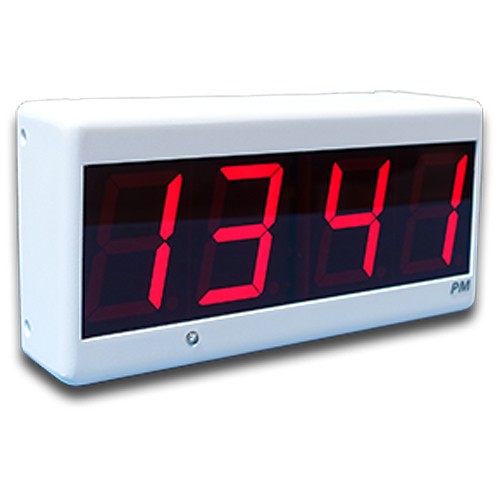A sleek, white digital alarm clock, resembling a brick in shape, is positioned at an angle facing towards the right. The front of the clock features a large black display with bright red digital numbers reading "13:41". Below the numbers, the letters "p.m." are displayed in black, indicating the time of day. The clock appears to be made from plastic and showcases a minimalist design. On the left side of the clock, there are two small holes, which could either be screw holes or decorative elements.